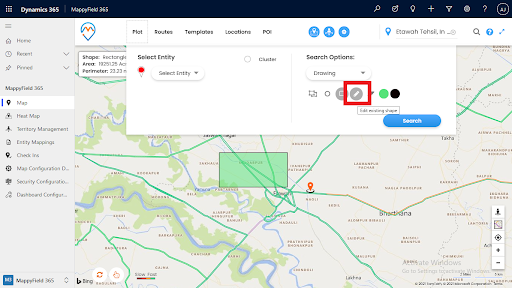Screenshot of a detailed map interface within a Dynamics 365 application. At the top left of the screen, partially visible text indicates that this is a Dynamics 365 map feature. A vertical menu on the left shows various options, with the "Map" option currently selected. Overlaying the map is a pop-up window titled "Select Entity," featuring selectable options on its left side. The right half of the pop-up is dedicated to "Search Options," currently set to "Drawing." Due to the small font size, the exact wording is challenging to decipher. A prominent blue "Search" button is located at the bottom right of this pop-up window. 

On the map itself, a green shaded rectangle highlights a specific area, adjacent to which a red map pin is placed. Towards the right of this green area, partially legible text appears, which seems to read "Shadiana," though the exact name is unclear due to the tiny and blurred text. The map interface provides a comprehensive set of tools for users to interact and search within the map boundaries efficiently.